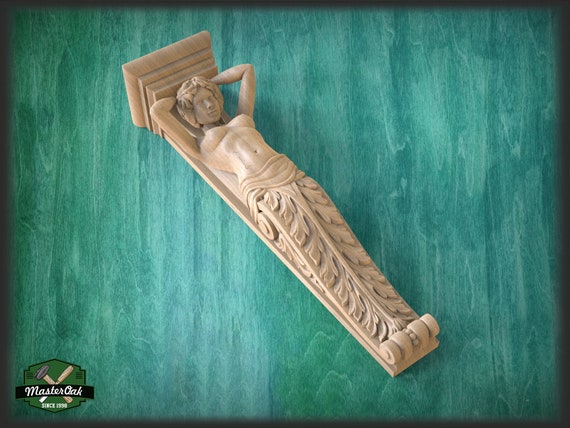This photograph showcases an intricately carved wooden sculpture, set against a teal-colored wood grain background, framed with a black border. In the bottom left corner, a green logo displaying a hammer crossed with a chisel and the words “Master Oak Since 1999” is prominently featured. The sculpture itself is designed as a pillar with a detailed depiction of a woman with short hair, lying down with her arms resting behind her head, and her torso unclothed. Her lower body is modestly covered with a cloth, and below the figure, the pillar transitions into a beautifully crafted foliage leaf pattern. The combination of craftsmanship and artistic detail creates a visually compelling piece.